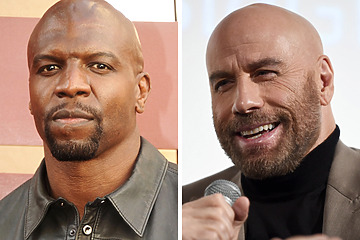This is a side-by-side collage featuring two different actors. On the left, there's a close-up image of Terry Crews, an African-American actor known for his muscular physique. He is bald with a goatee and has a stern expression. He is dressed in what appears to be a leather jacket, standing against a peach or salmon-colored backdrop, likely taken during a press event. On the right, there's a close-up image of John Travolta, a white actor with a bald head and a prominent beard. He is smiling and holding a microphone, wearing a brown suit jacket over a black turtleneck. This collection captures two well-known figures in contrasting yet complementary poses and expressions.